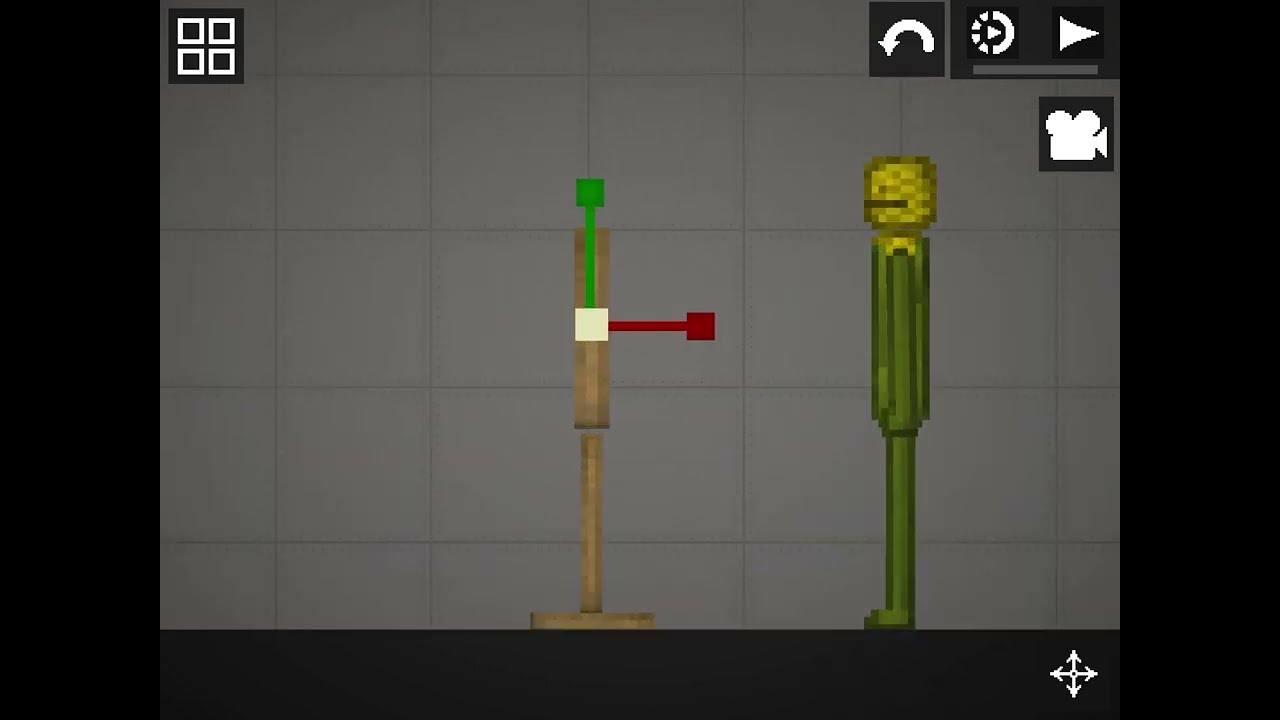The image appears to be a pixelated screenshot of an old, simplistic-looking video game. Set against a black background, the scene centers on two stick-figure characters standing on a gray, tiled platform. The character on the left resembles a wooden stick figure with a green square head, a green shaft extending upward, and a red appendage extending forward horizontally. This figure is depicted as interacting with another stick-figure character on the right, which has a yellow, robot-like head with a brown slit for a mouth, a green body, and matching green legs. The surrounding interface includes a quadrant box with white squares in the upper left corner and a set of black buttons on the upper right, featuring icons for navigation (a curved arrow to go back and a play button), and a film camera symbol. The scene is framed by black rectangular borders on both sides.